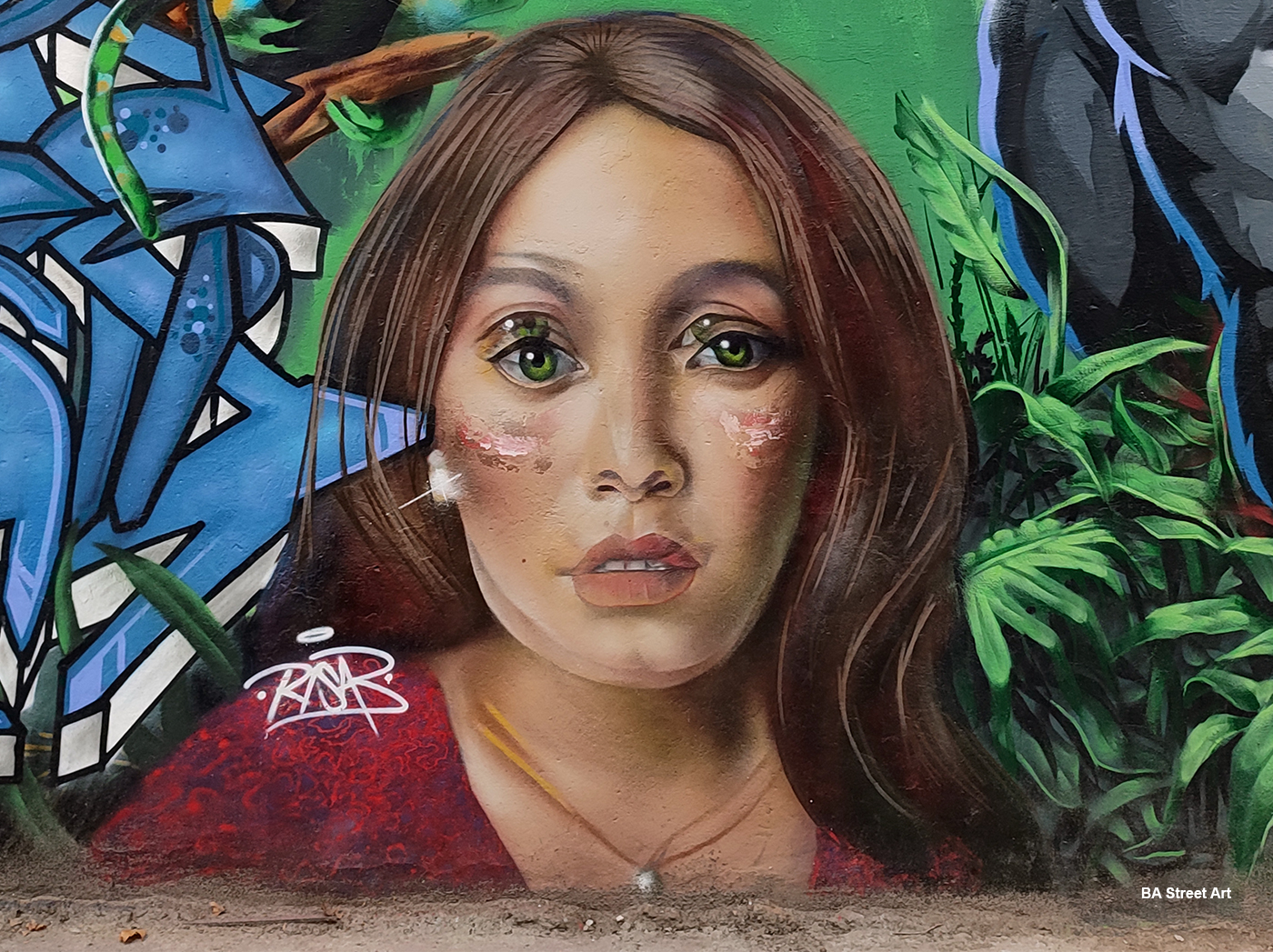The mural, a striking piece of BA Street Art, portrays a hyper-realistic and slightly jarring image of a woman with warm brown hair falling around her shoulders and olive skin. Her green eyes are duplicated, creating a dizzying effect reminiscent of a blurred motion photograph. She wears pink cheeks, pink lipstick, and a red dress, complemented by a gold necklace featuring a silver pendant at its center. The incomplete look of the necklace and the disorienting eyes add an almost AI-generated feel to the piece.

To her left, blue graffiti with arrow-like shapes and lines stands out against the vibrant colors of the mural. Just above the crown of her head, a green wall, brown branch, and painted water with black rocks create a layered backdrop. On her right, green plants grow upwards, reaching close to her head, and gray rocks outlined in blue add to the natural elements in the artwork. The ground below is depicted with brown soil, grounding the mural.

The artist's signature, which appears to read "Risa," is inscribed in white on her left shoulder, while at the bottom right corner, the text "BA Street Art" is prominently featured, indicating the mural's origin. This intricate work captures a surreal blend of natural and abstract elements, creating a mesmerizing visual experience.